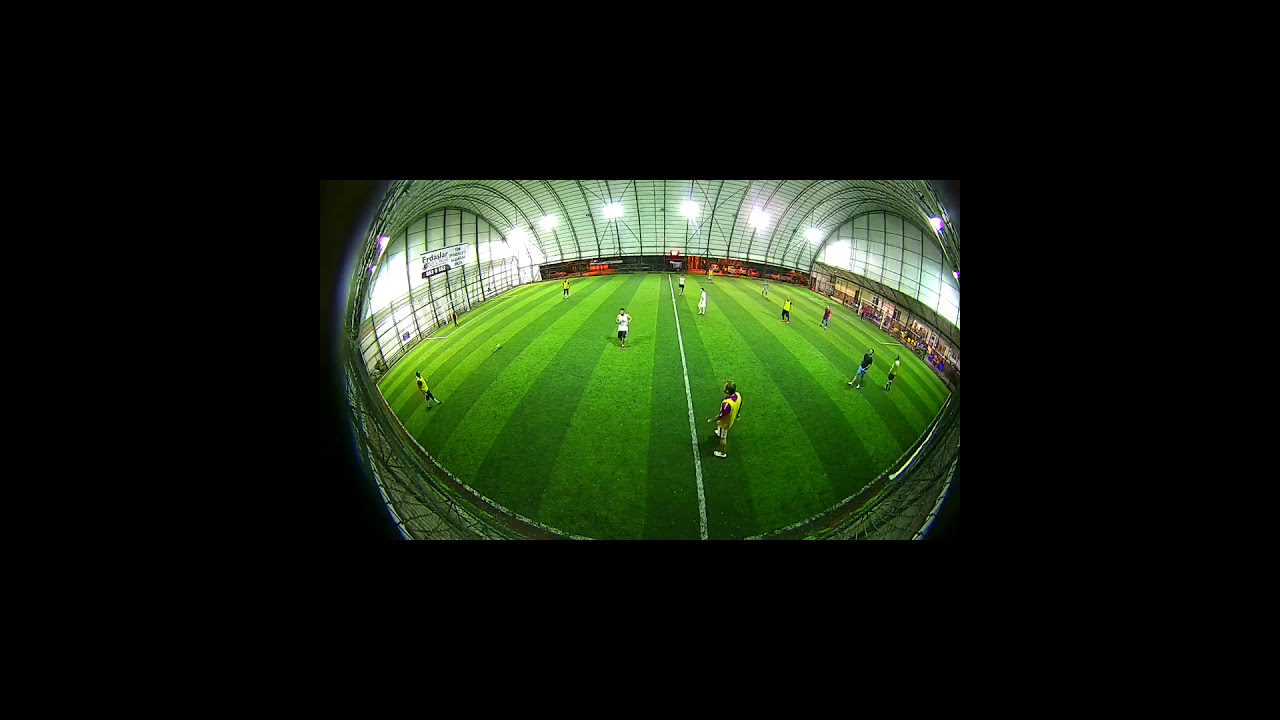This captivating indoor soccer field photograph exhibits several detailed elements, framed by a thick, black border that occupies much of the top, bottom, and sides. At the heart of the image, amidst the panoramic distortion, is a vividly green and white striped field, marked by a bright white line dividing its center. Players clad in diverse colors—yellow, white, red, purple, gray, and tan—are engaged in the game, positioned centrally within the frame. The field is enclosed within an arched, airplane hangar-like dome, supported by steel columns, and adorned with lights that illuminate the interior. To the right of the field is a small bleacher area crowded with spectators, while the left side lacks any seating. Despite the panoramic nature of the shot making the relative positions somewhat hard to discern, the overall composition clearly portrays an active indoor sports arena.